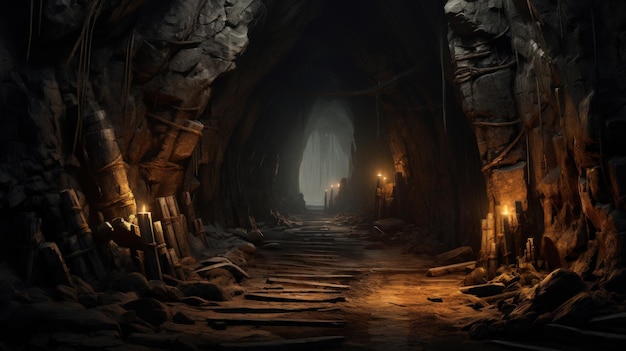The image is an intricately illustrated digital drawing of a large, dimly-lit cavern. The scene features horizontal wooden planks laid out on the ground, forming a makeshift pathway that guides the viewer's eye deeper into the cave. To the left and right of this walkway, various bundles of wood and stone pseudo-columns, bound together for stability, line the walls. Sparse, flickering candlelight casts an amber-yellow glow, with one candle prominently positioned close to the viewer on the left side and several more extending further down the right, illuminating the cavern's features. The rocky walls, painted in shades of gray and dark brown, rise upwards, festooned with hanging vines and ropes, adding texture to the scene. The cavern extends to another opening in the distance, framed by hanging formations and shrouded in a mysterious fog, hinting at further unexplored depths.